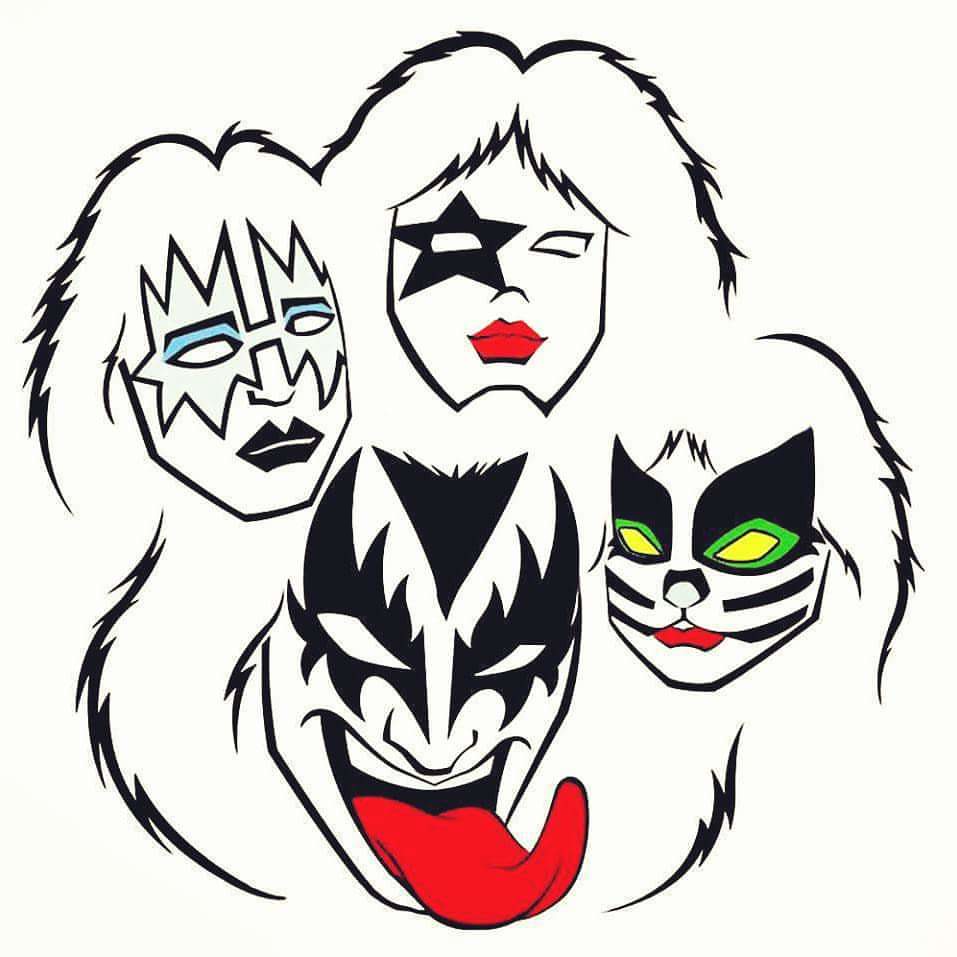This image is a detailed line drawing on a white background, using black ink, reminiscent of the rock band KISS, depicted in their iconic makeup. The four faces are centrally grouped together and outlined in black, lending a sticker or tattoo-like quality to the design.

At the bottom, there is a figure characterized by a long jaw and a distinctive, red tongue sticking out, curled at the tip. This face features a bat-like mask around the eyes with four jagged points at the top, several below the eyes, and one along the nose, and an inverted black V representing hair.

Moving counterclockwise to the three o’clock position, the next face resembles a black cat with a red lower lip, small cat-like nose, two cheek stripes, and defined bangs with longer hair. The area above the eyes is heavily black, leading to points, with inner sections colored green fading to yellow.

At the twelve o’clock position on top, there is a face with longer hair parted in the middle, a bold black star around the right eye, and prominent red lips.

Finally, at the ten o’clock position, the figure has light blue eyeshadow above the eyes, intricate black markings, a vertical stripe from the nose up, a horizontal bar across the nose, and black lipstick completing the look.

The drawing varies in line weight to provide depth and detail, especially in the hair which is rendered in jagged lines. The overall black and white composition, punctuated by selective color details (red tongue, green and yellow eyes, red lips, and blue eyeshadow), captures the essence of each band member’s unique KISS persona.